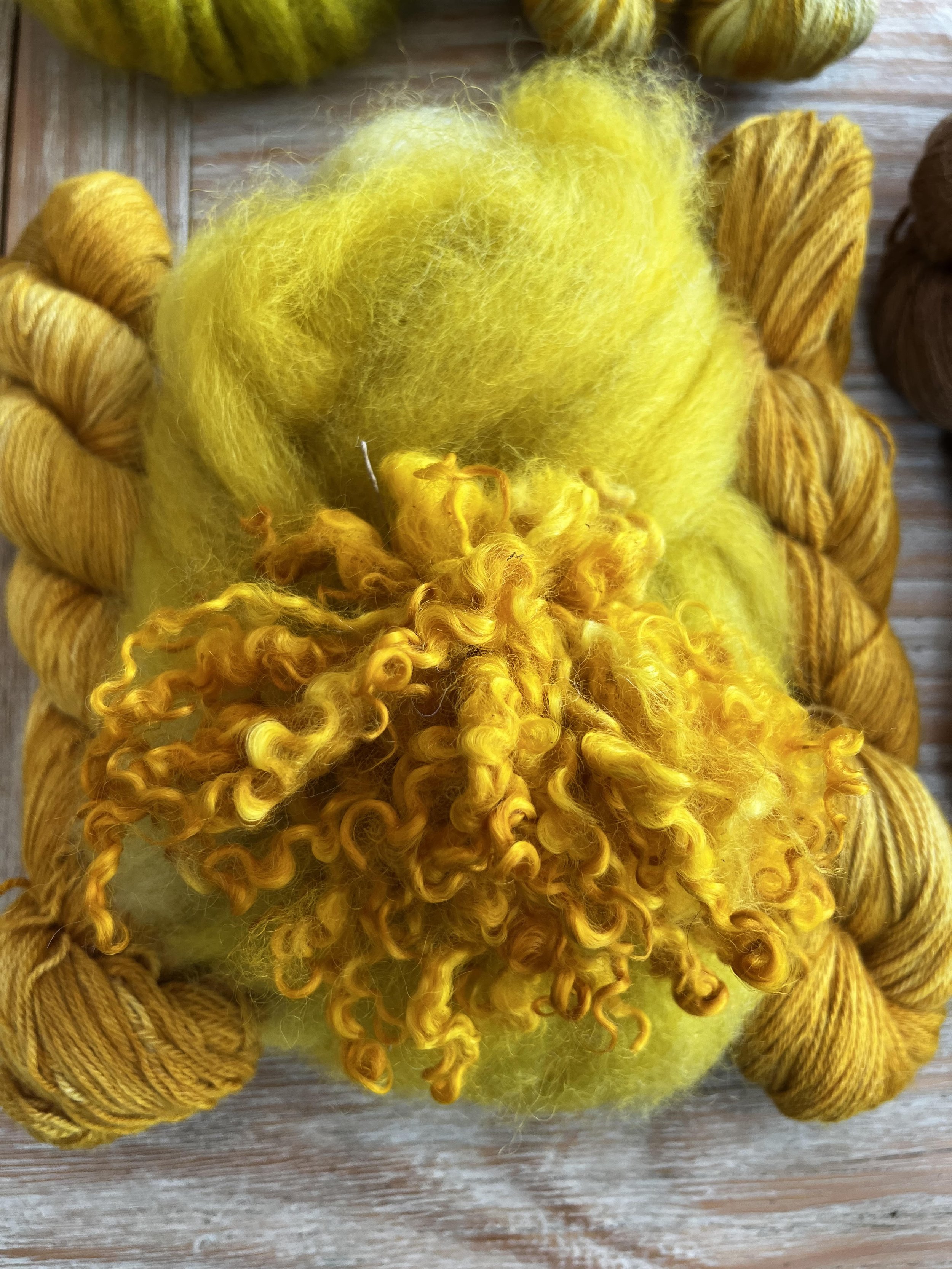The image features an organized arrangement of yarn, predominantly in shades of gold and yellow. At the center, there is a fluffy, bright yellow material that appears soft and plush, resembling filler or stuffing. This central fluffy section is flanked by two bundles of yarn on either side. Above the fluffy center, there is a darker yellow yarn twisted into tight, hair-like curls. The entire setup is placed on a wooden tabletop with a faded, lighter wood texture. Surrounding the central fluffy bundle, additional clumps of yarn can be seen, with some positioned towards the top and sides of the image. Despite the varied interpretations, the focus remains clearly on this intricate display of different yarn materials, with colors including white, light tan, golden mustard, yellow, and light green. The photograph emphasizes the textures and organization of the yarn without any accompanying text, highlighting the craft materials in a detailed and deliberate composition.